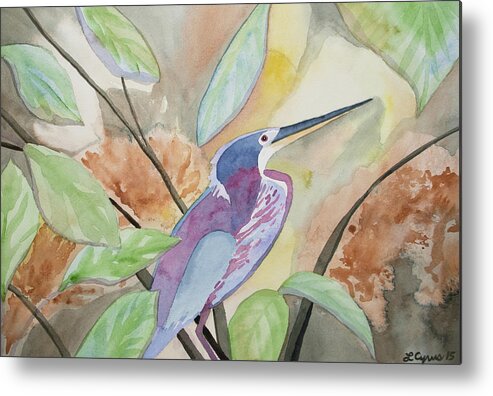This painting features a striking bird perched on a dark brown tree branch, amidst a lush environment of green leaves and diverse background hues. The artist has signed the canvas, which seems to read "L... [indistinct] Cyrus 15." Executed in watercolors or pastels, the painting captures the bird in a profile view with a long beak, the top of which is a dark blue and the bottom a yellowish tone. The bird's head is navy blue with red eyes and features a strip of light blue along the side. Its body showcases an intricate blend of purple and blue feathers, complemented by light blue wings and purple legs. The composition is set against a white backdrop framed by a thin black line, with background tones speckled in light brown and hints of orangish color. The scene exudes a soft, almost geometric style, making it an exquisite and delicate interpretation of avian beauty in its natural habitat.